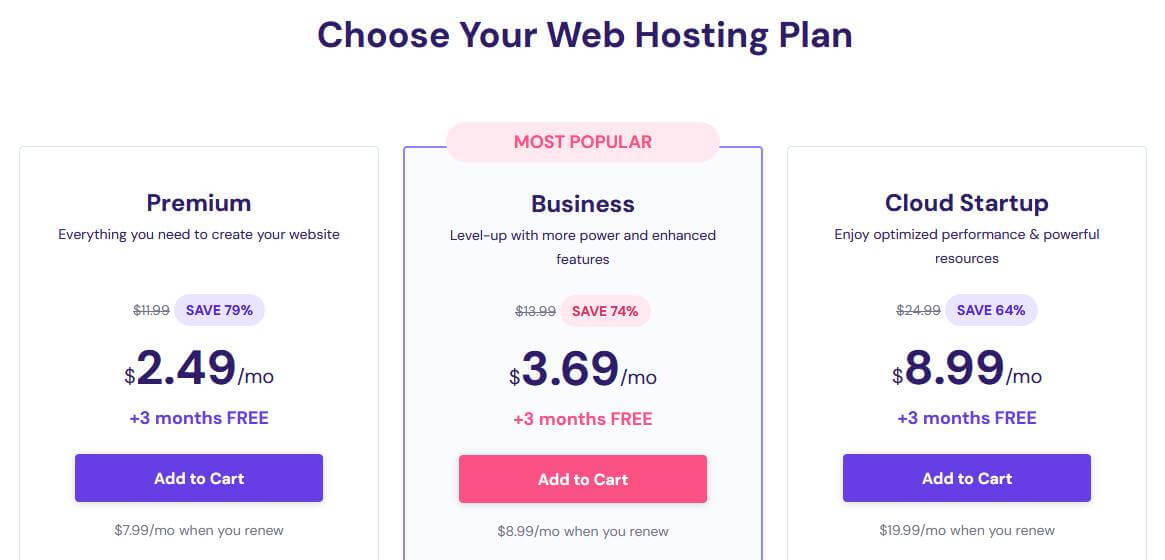The image is a screenshot featuring a predominantly white background with a central heading at the top that reads, "Choose Your Web Hosting Plan." The content is organized into three columns, each presenting a different web hosting option.

**First Column (Left):**
- **Title:** Premium
- **Description:** "Everything you need to create your website."
- **Pricing:** Originally $11.99, now discounted by 79% to $2.49 per month, plus three months free.
- **Button:** A rectangular purple button labeled "Add to cart."
- **Renewal Price:** $7.99 monthly.

**Second Column (Middle):**
- **Heading:** "Most Popular" in a pinkish hue.
- **Title:** Business
- **Description:** "Level up with more power and enhanced features."
- **Pricing:** Originally $13.99, now discounted by 74% to $3.69 per month, plus three months free.
- **Button:** A rectangular pink button labeled "Add to cart."
- **Renewal Price:** $8.99 monthly.

**Third Column (Right):**
- **Title:** Cloud Startup
- **Description:** "Enjoy optimized performance and powerful resources."
- **Pricing:** Originally $24.99, now discounted by 64% to $8.99 per month, plus three months free.
- **Button:** A rectangular purple button labeled "Add to cart."
- **Renewal Price:** $19.99 monthly.